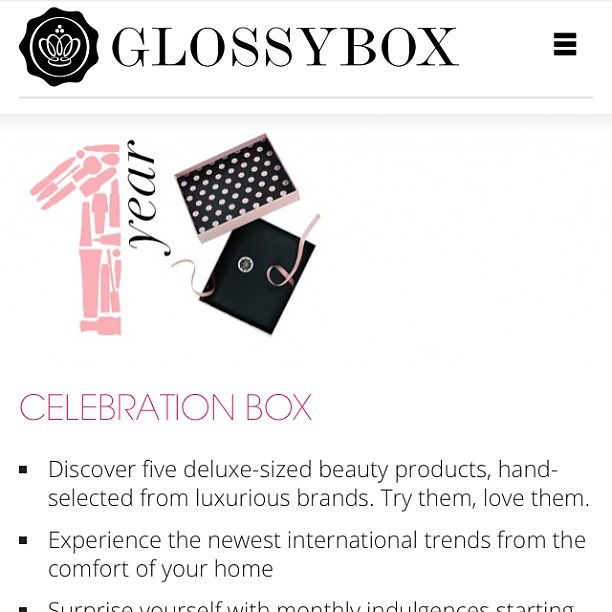The image is a screenshot from the Glossy Box website, showcasing a celebratory offering. At the top, the header features a rounded emblem on the left with a white crown inside a black beveled stamp, and the word "Glossy Box" in black font to the right, followed by three horizontal dashes. Below this header, on the left, the phrase "1 Year" is prominently displayed, with the number 1 creatively formed out of pink silhouettes of various makeup products like mascara, brushes, and nail polish, arranged vertically next to the word "YEAR" in black font. Adjacent to this, there are two small boxes, one pink with a black interior and the other black, possibly representing a makeup case or cover. Further down, large pink text reads "CELEBRATION BOX," followed by three black bullet points. The first bullet point states: "Discover five deluxe size beauty products hand-selected from luxurious brands. Try them, love them." The second reads: "Experience the newest international trends from the comfort of your home." The third bullet point appears to be partially cut off, but it suggests: "Surprise yourself with monthly indulgence starting..." All of this is set against a clean white background.